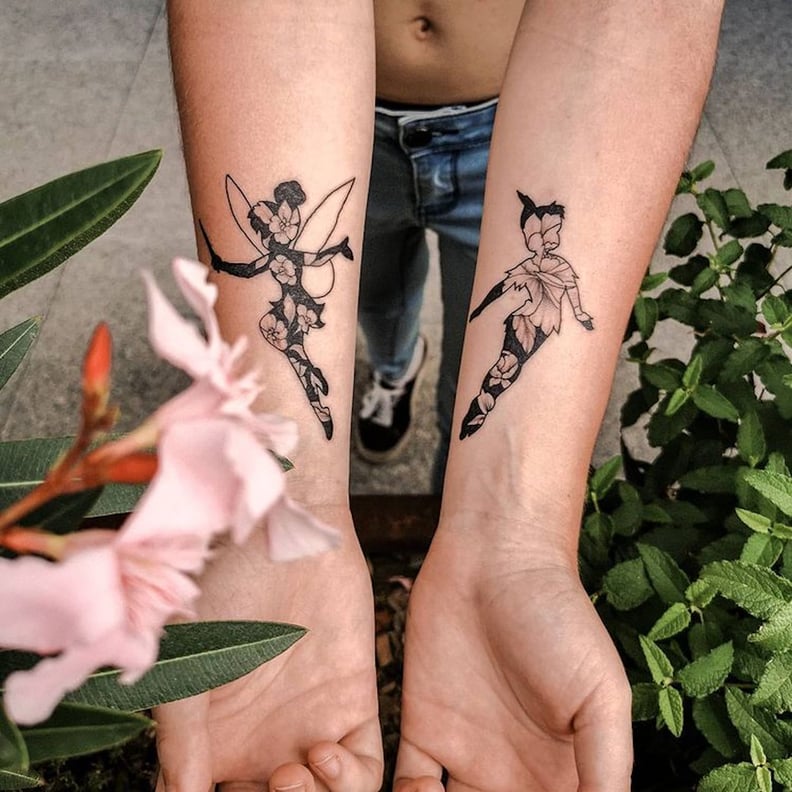The image showcases the forearms and wrists of a shirtless person wearing blue denim jeans and black sneakers, standing on a gray cement surface. Their arms, extended forward, reveal intricate black tattoos of Tinkerbell on the left arm and Peter Pan on the right arm. Both whimsical characters are depicted in flight, filled with intricate floral patterns, with Tinkerbell's wings and bent knees and Peter Pan's feathered hat adding to their dynamic poses. The background features a lush array of real flowers, with vibrant orange and pink blossoms accompanied by green leaves on the left side, and lighter green leaves on the right side. The person's skin, visible from the belly button down, is a pink-tan hue, and some of their fingers are slightly curled and partially visible in the frame. The image contains no text.